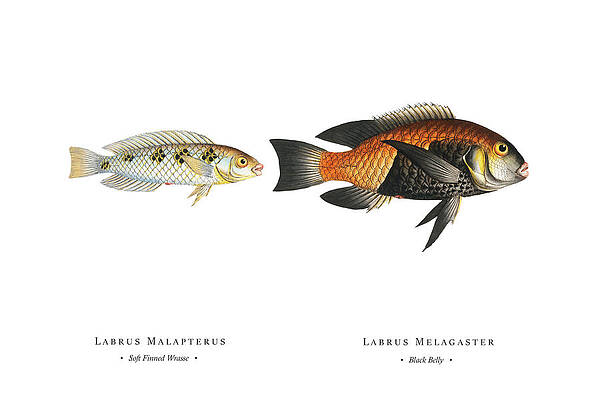The digitally generated educational image showcases two fish side by side against a red background. On the left, the smaller fish is primarily white with golden hues and black star-like scales along its back. It features long fins on one side and shorter fins on the other. This fish is labeled "Labrous Marupterus" and is described as soft-finned. The larger fish on the right has a more robust body adorned with a striking combination of golden-brown scales on the upper part and a black belly. Its fins are long and sharp, predominantly black, with occasional white touches. The face is grayish with light, orangish lips and an eye ringed with orange. This fish is labeled "Lazarus Melagaster, black belly." Both fish are depicted in side view, highlighting their distinctive colors and detailed anatomical features.